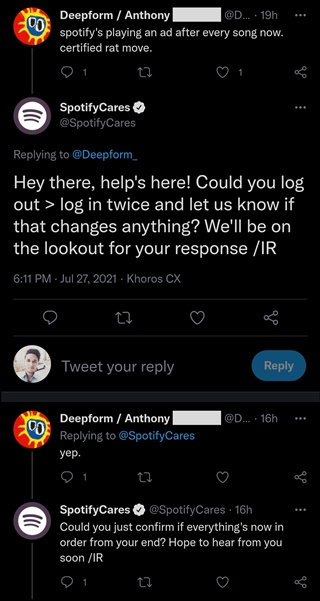**Detailed Caption:**

The image is a screenshot of a Twitter conversation captured on a mobile device, likely an Apple or Android phone. The screenshot displays a thread involving a user and the official Spotify Cares support account. The initial tweet by the user, named "Deep Form Anthony" (with part of the name obscured), complains: "Spotify is playing an ad after every song now. Certified rap move."

Spotify Cares, a verified account, promptly responds: "Hey there, Helps here. Could you log out, log in twice, and let us know if that changes anything? We'll be on the lookout for your response. /IR" This response is timestamped at 6:11 PM on July 7, 2021, and sent from Coros CX. 

Subsequently, "Deep Form Anthony" replies with a brief "Yep." This reply is sent approximately three hours after the original tweet. Following this, Spotify Cares responds again, requesting confirmation: "Could you just confirm if everything's now in order from your end? Hope to hear from you soon. /IR" The screenshot indicates that there is a reply to this last tweet from the user, but it is not visible in the captured image.